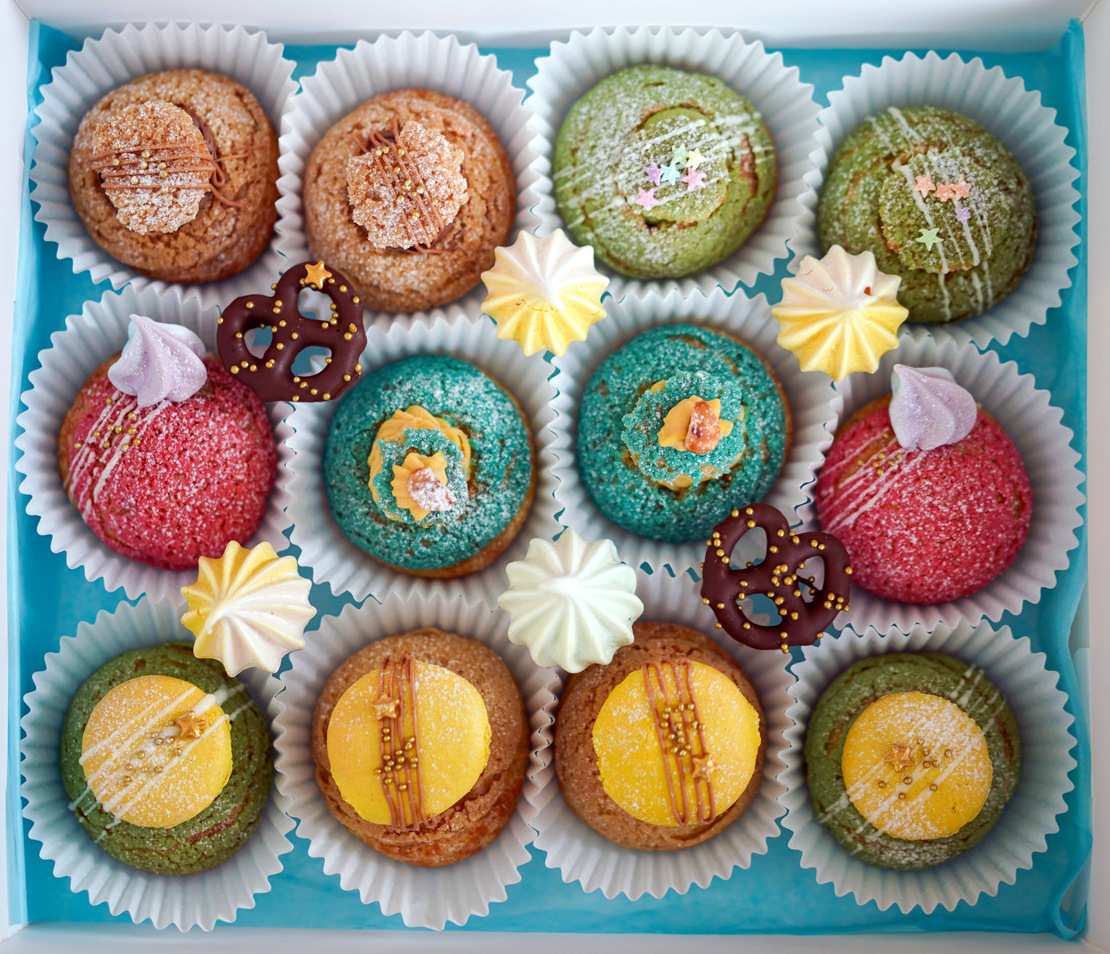The image is an overhead shot of a white box lined with a blue liner, filled with 12 assorted macaroons, each nestled in white muffin papers. There are two macaroons of each flavor and color: brown, green, pink, blue, green with yellow fondant, and brown with yellow fondant. The macaroons are arranged in three rows of four. Two chocolate-covered pretzels, adorned with yellow specks of icing, are strategically placed atop the white muffin papers, separating the cookies. Surrounding the macaroons, there are buttermints used as additional decoration. The macaroons and pretzels are elaborately decorated with various frostings and fondant pieces, including stars and drizzles, adding a vibrant and festive touch to the display.